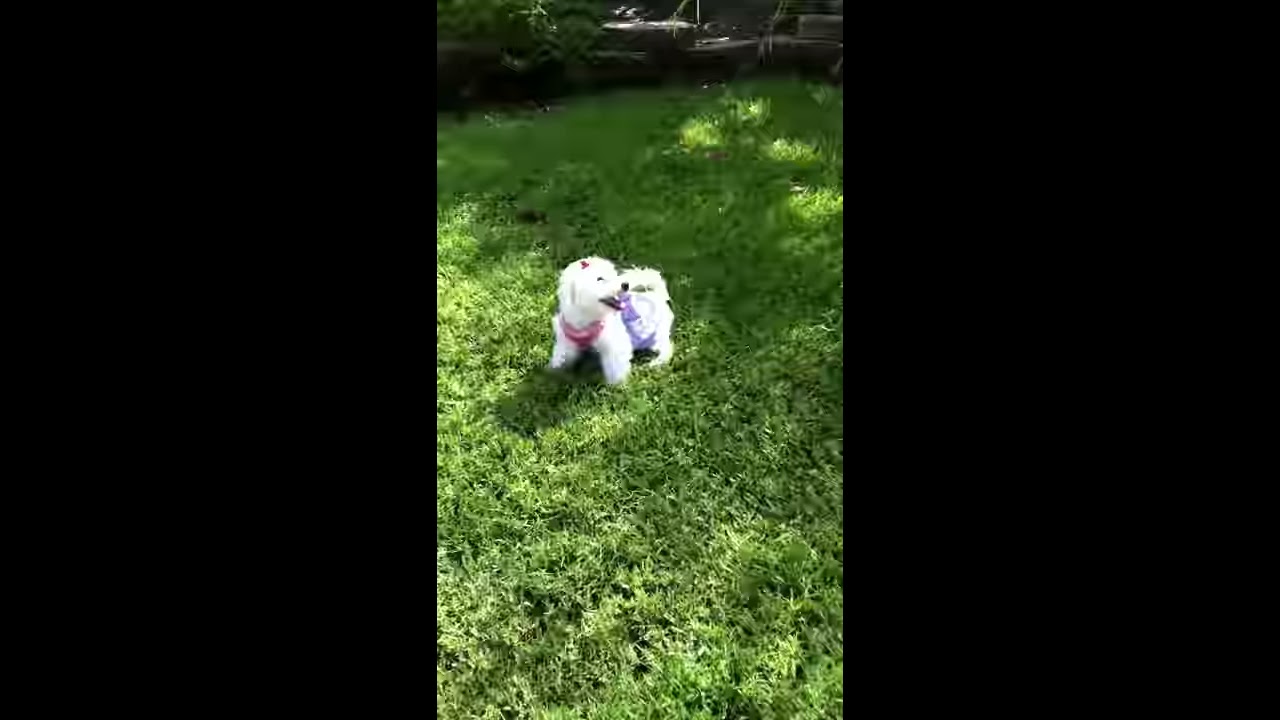In the image, there is a small, fluffy, white dog standing in the center of a slightly overgrown, green grassy yard. The dog appears to weigh between 10 to 20 pounds and is energetically wagging its tail, giving a joyful impression. Adorning the dog is a pink scarf around its neck along with additional decorations: a possible pink skirt around its back and a bow or hat on its head. The dog’s mouth is open, suggesting it's in a lively mood, possibly reacting to something off to its left, maybe its owner. In the background, there are a couple of trees, some seats or a swing set, and what looks like a fence with overgrown grass, creating a laid-back outdoor scene. Despite the low quality and heavy compression of the photograph, the dog's happy demeanor is clearly visible as it enjoys its time in the yard.